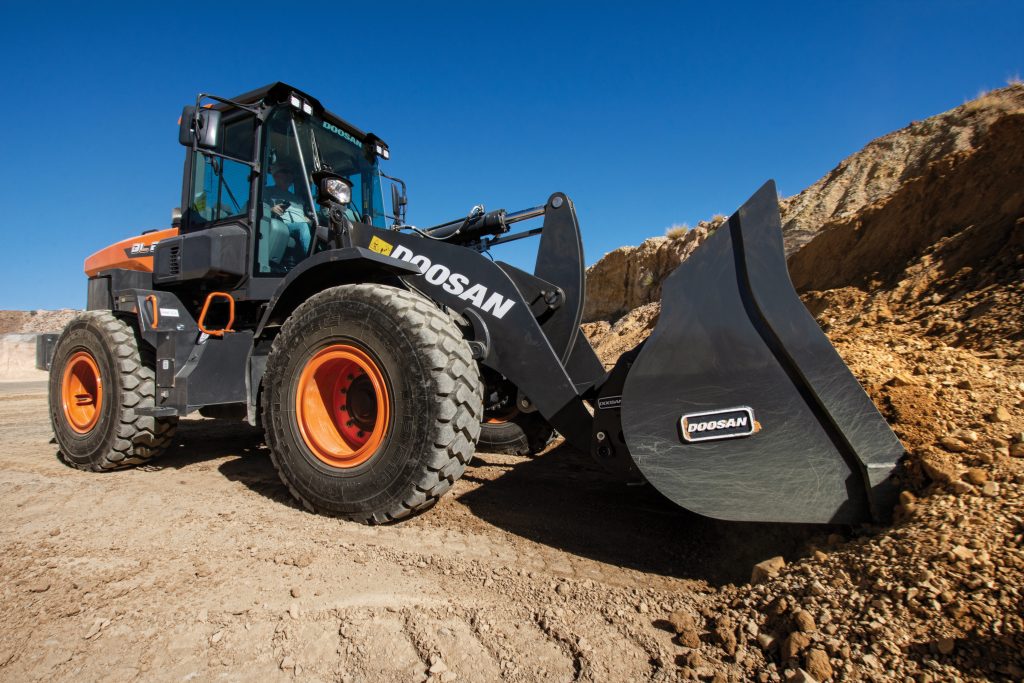The image portrays a close-up, outdoor daytime photograph of a Doosan front loader in action, set against a clear, cloudless sky. The vehicle, which is mostly black with bright orange rims on its large, dust-covered wheels, is captured from the side as it scoops up a substantial load of dirt. It appears to be positioned on level ground, likely within a quarry, and no other vehicles or background elements are visible. The front loader, which is almost brand new and bears the Doosan emblem on its side and bucket, is operated by a driver dressed in blue jeans and a white button-down shirt. Additional features visible on the vehicle include a side mirror and an orange handle near the driver's cabin. The clean and pristine state of the loader suggests this image might be intended for publicity or marketing purposes.